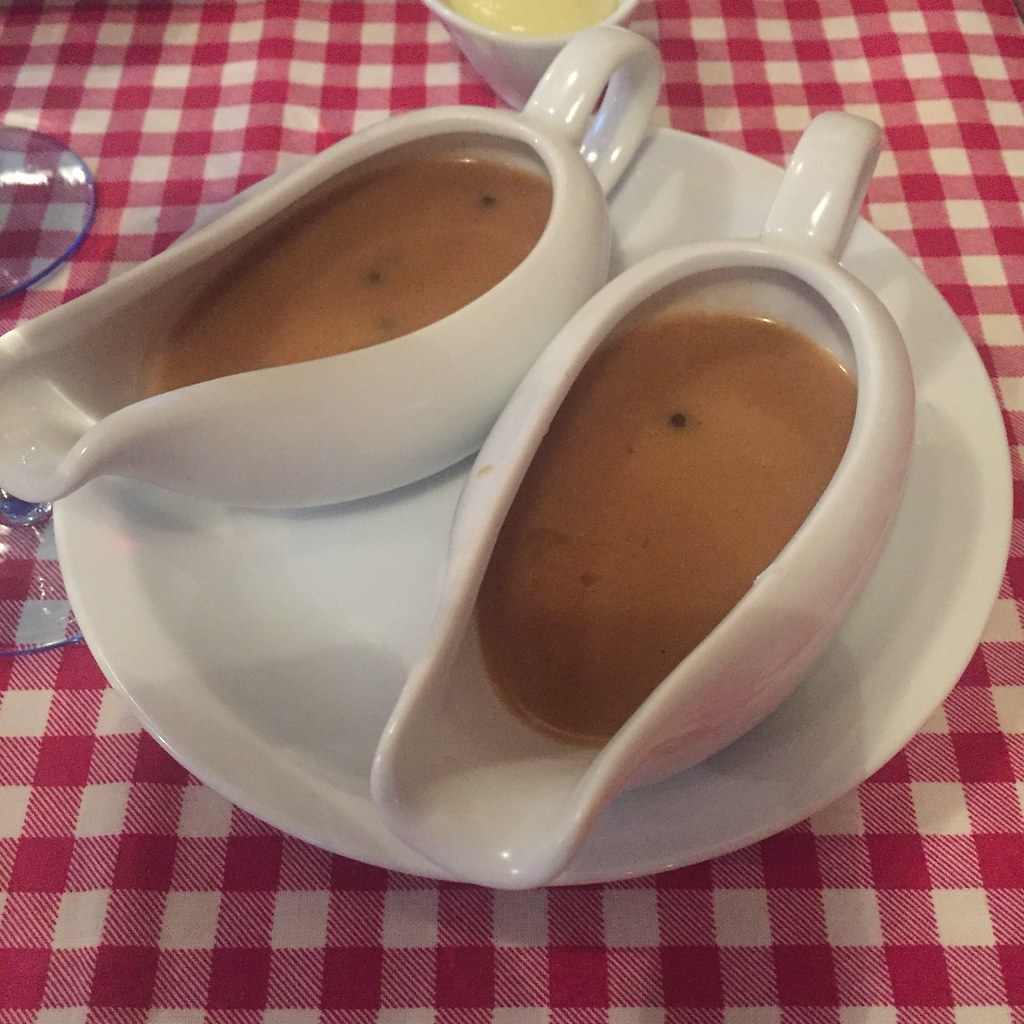The image features two white gravy boats positioned on a single white plate, each filled with a tan, viscous gravy speckled with black peppercorn-like bits. The plate is situated on a red and white checkered tablecloth, reminiscent of an Italian restaurant setting. Just behind the gravy boats, there is a white dish holding a yellow or beige creamy substance, possibly butter or mayonnaise. On the left, part of a blue-tinted, see-through glass plate is visible. Additionally, the bases and stems of stemmed glasses are partially seen on the left side, slightly cut off by the frame of the image.